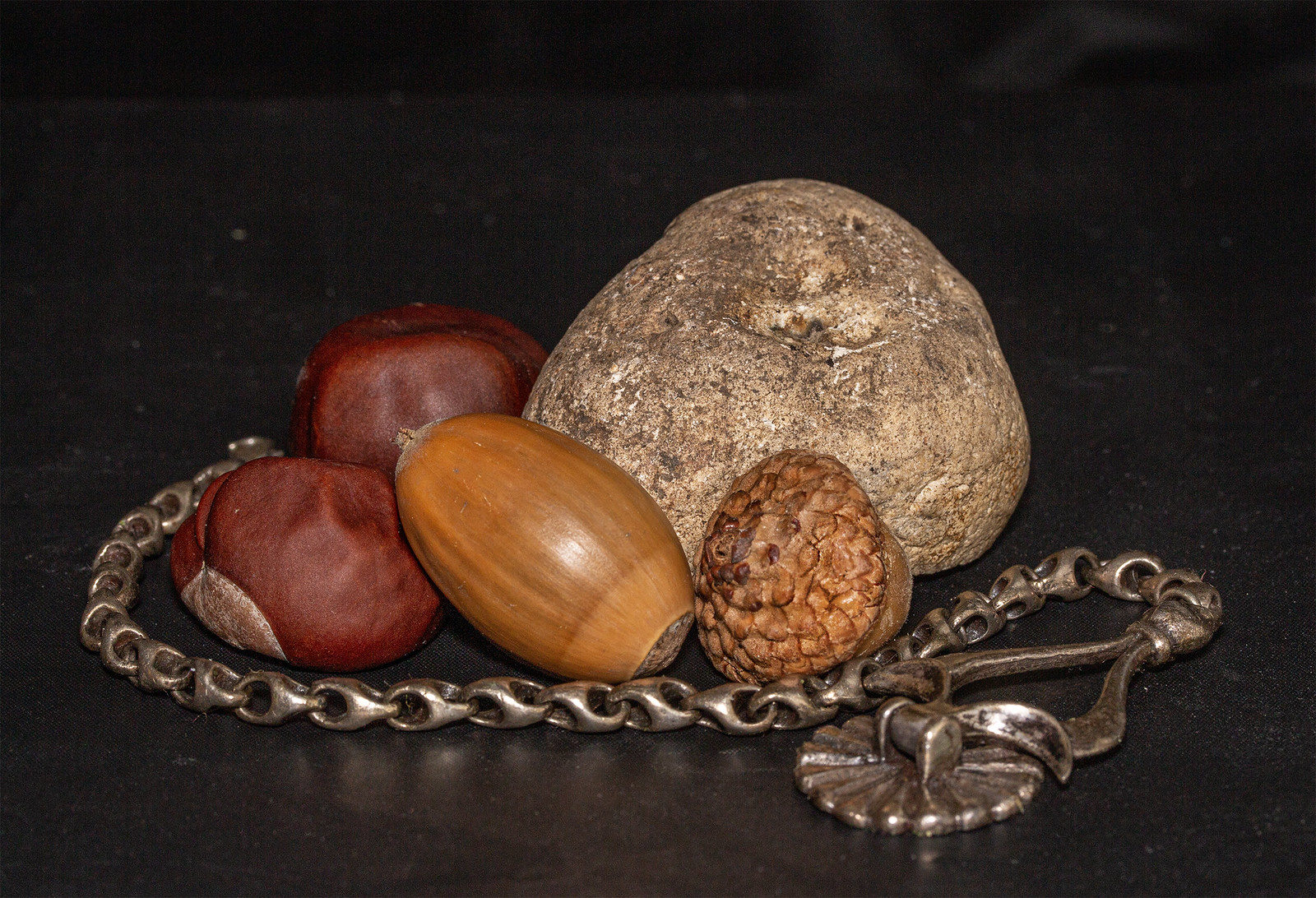In this artistic photograph set against a black background, a collection of nuts and a prominent rock are meticulously arranged. The large rock, about six inches tall, is predominantly dark tan with patches of dirt and lighter spots with small indentations at the top, giving it a slightly weathered appearance. In front of the rock, there are two buckeyes - reddish-brown and smooth, positioned next to one another, almost like miniature dark apples. Nearby, a hazelnut, with its characteristic smooth, light brown surface marked by darker brown stripes, tilts slightly towards the upper left, evoking the look of a pecan. An acorn with a brown cap lies on its side, adding to the variety of textures and shapes. Encircling the entire arrangement is a heavy, thick-linked silver chain that wraps around the rock and the nuts. At one end of the chain, a prominent silver disc pendant - about two inches long - gleams subtly, adding an industrial touch to the earthy composition.